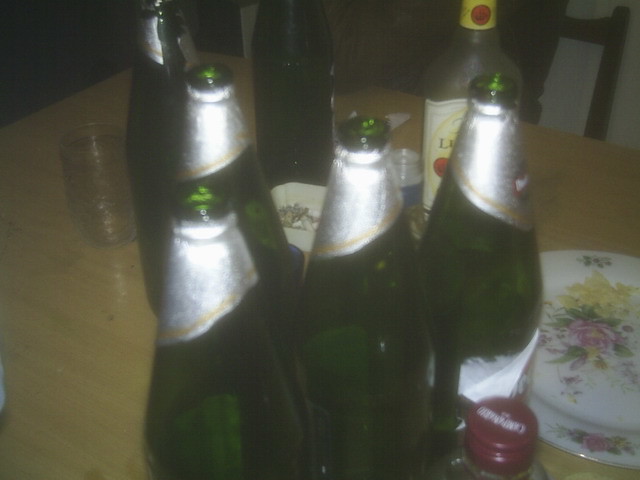The photograph is a slightly blurred, vintage image depicting a light brown, wooden table, likely in a restaurant. On the table, there are seven bottles, mostly green wine bottles with the silver accent around their tops. At least four of these bottles have their corks removed. Among the bottles, one toward the right has a distinctive square label featuring a white and yellow design with a red circle, possibly indicating a different type of drink. Another, darker bottle is also partially visible. To the right, there's a red-capped bottle with indistinguishable white writing. A small tumbler glass sits on the left side of the table.

In the right bottom corner rests a white plate adorned with pink floral designs in the center and along the edges, likely a coaster. Additionally, a small white ashtray containing put-out cigarettes is near the center of the table. The background of the image reveals parts of a dark-colored kitchen chair on the right and a shadowed area to the upper left. The entire scene conveys an old-world charm, capturing what appears to be remnants of a social gathering.